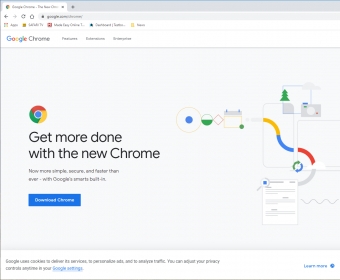This is a detailed caption following the cleanup and reformulation process:

The screenshot captures the introductory page of Google Chrome on a computer screen. The background is primarily white with accents of light gray. At the center, prominently displayed in black lettering, is the message: "Get more done with the new Chrome." Although the text beneath this headline is not fully legible, it is clear that it contains additional information. Below the text, a prominent blue button with white lettering invites users to "Download Chrome." 

On the right side of the page, there is a visually engaging section featuring an array of images resembling a science experiment. These images combine various shapes and colors associated with Chrome's branding: yellow, blue, red, and green. The shapes include circles, squares, and a diamond, interconnected to symbolize the elements that make up Google Chrome. Towards the bottom, there is an illustration of a webpage, depicted in white with gray elements, adding to the visual narrative of the browser's design and functionality.